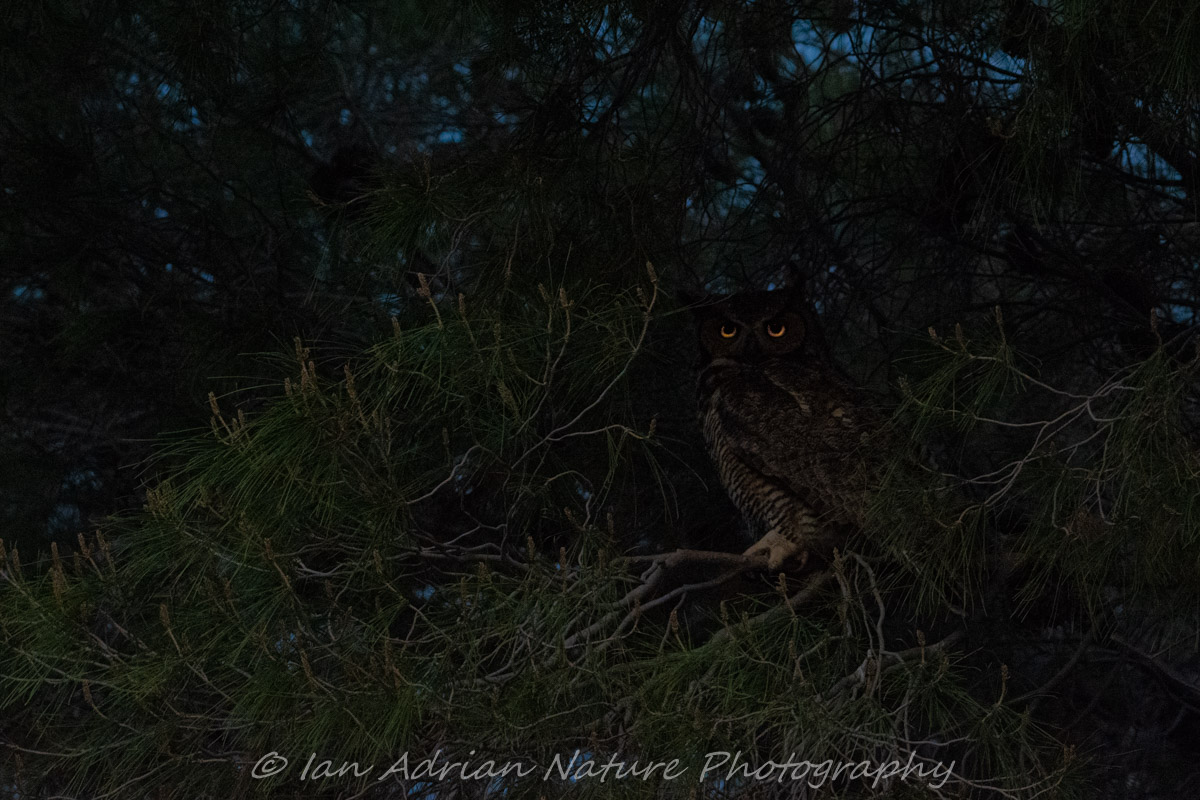The image depicts a dense forest scene, likely photographed in the evening or nighttime, dominated by thick, intertwining branches that obscure the trunk, creating a sense of depth and mystery. Amidst the darkness, a striking owl with dark brown and black feathers is perched on a branch, its sharp talons clearly visible. The owl's head is turned towards the camera, revealing its piercing yellow eyes that reflect light like two glowing half-moons, adding an eerie glow to the scene. A small patch of blue sky peeks through the dense foliage, offering a slight contrast to the predominantly dark background. At the bottom center of the image, a watermark in white letters reads "I am Adrian Nature Photography," marking the photo's authenticity.